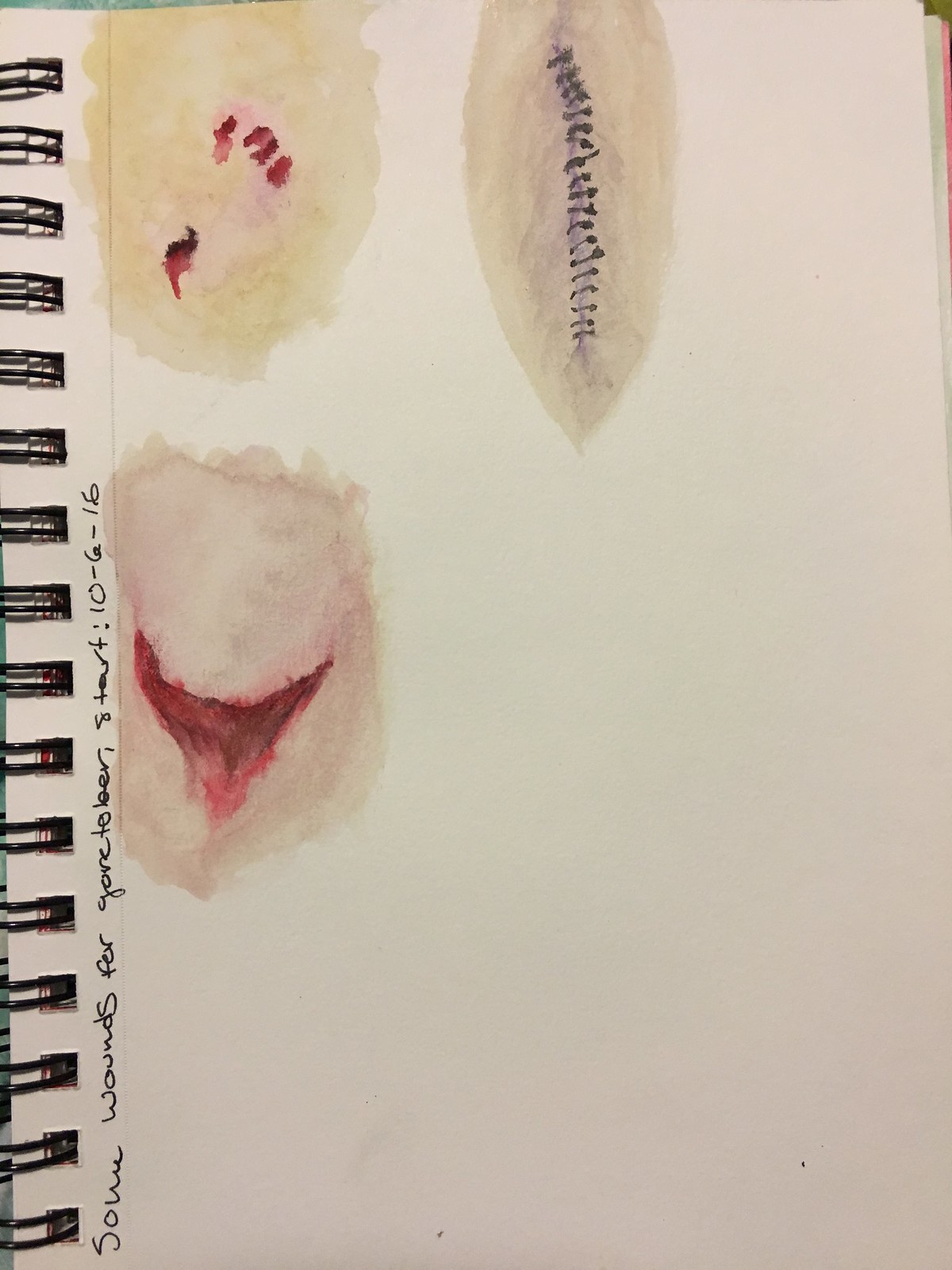The image is a detailed color photograph of an opened, ring-bound sketchbook or notebook. The notebook is positioned so that its black spiral binding is visible on the left side of the image. The topmost page, likely of construction paper, is predominantly off-white, and beneath it, various colored pages in blue, green, and pink can be seen.

Along the margin beside the spiral binding, written vertically from bottom to top, is the text "some wounds for Gortober, Start 10-6-16." The page features three small watercolor paintings arranged in two rows. The paintings depict realistic, flesh-colored wounds with intricate details. The top drawing shows a series of four bloody wounds in flesh tones, highlighted with bright reds representing cuts. Adjacent to this is a leaf-shaped wound with a grayish hue and black lines resembling stitches running down the center, slightly filled with purple along the stitch line. Below these, a drawing appears to delineate a gaping wound on a torso, characterized by its bloody, raw appearance. The vivid use of color and the meticulous detailing of these imaginary wounds give the notebook page a clinical and artistic appeal.